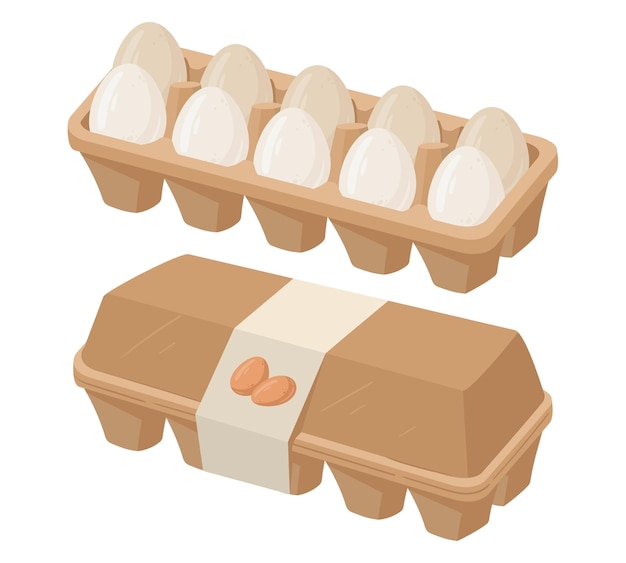A detailed illustration depicts a tan-colored cardboard egg carton, branded with a band that features an emblem of two eggs. The first part of the image shows the carton closed, displaying the logo prominently. The second part reveals the carton opened, showcasing 10 neatly arranged white eggs inside. The carton, designed to hold a dozen, is depicted with all objects upright, emphasizing the product's neat and organized presentation.